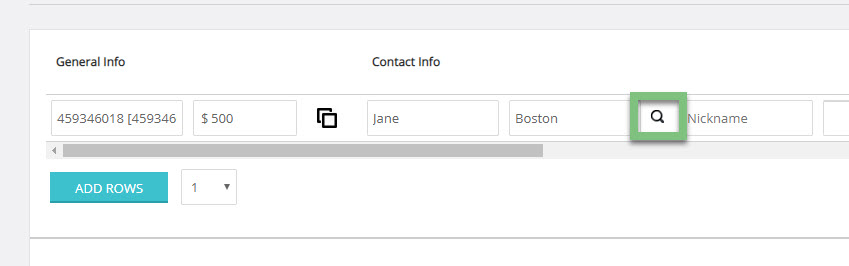The image displays a structured layout on a white background with a distinct gray border at the top and left edges. At the bottom, there is a thin gray line extending horizontally from left to right. In the top left section of the box, the 'General Info' section is prominently positioned. Adjacent to it towards the center is the 'Contact Info' section. 

Below these sections, a thin gray line divides them from the rest of the content. Towards the center of the box, there is a larger rectangle bordered in gray. Within this rectangle, the number "4593346018" is displayed centrally. Near it, a bracketed number "459346" is also visible.

To the right of this rectangle, there are sequentially aligned smaller boxes:
1. The first box on the right contains the text "$500."
2. Next to it, another box simply labeled "Chain."
3. Following this, a box labeled "Boston."
4. Adjacent to this, there is a green square enclosing a magnifying glass icon.
5. Finally, a box labeled "Nicknames" is positioned further to the right.

This detailed layout presents a methodical arrangement of information with specific sections and numerical details, enhancing clarity and organization.